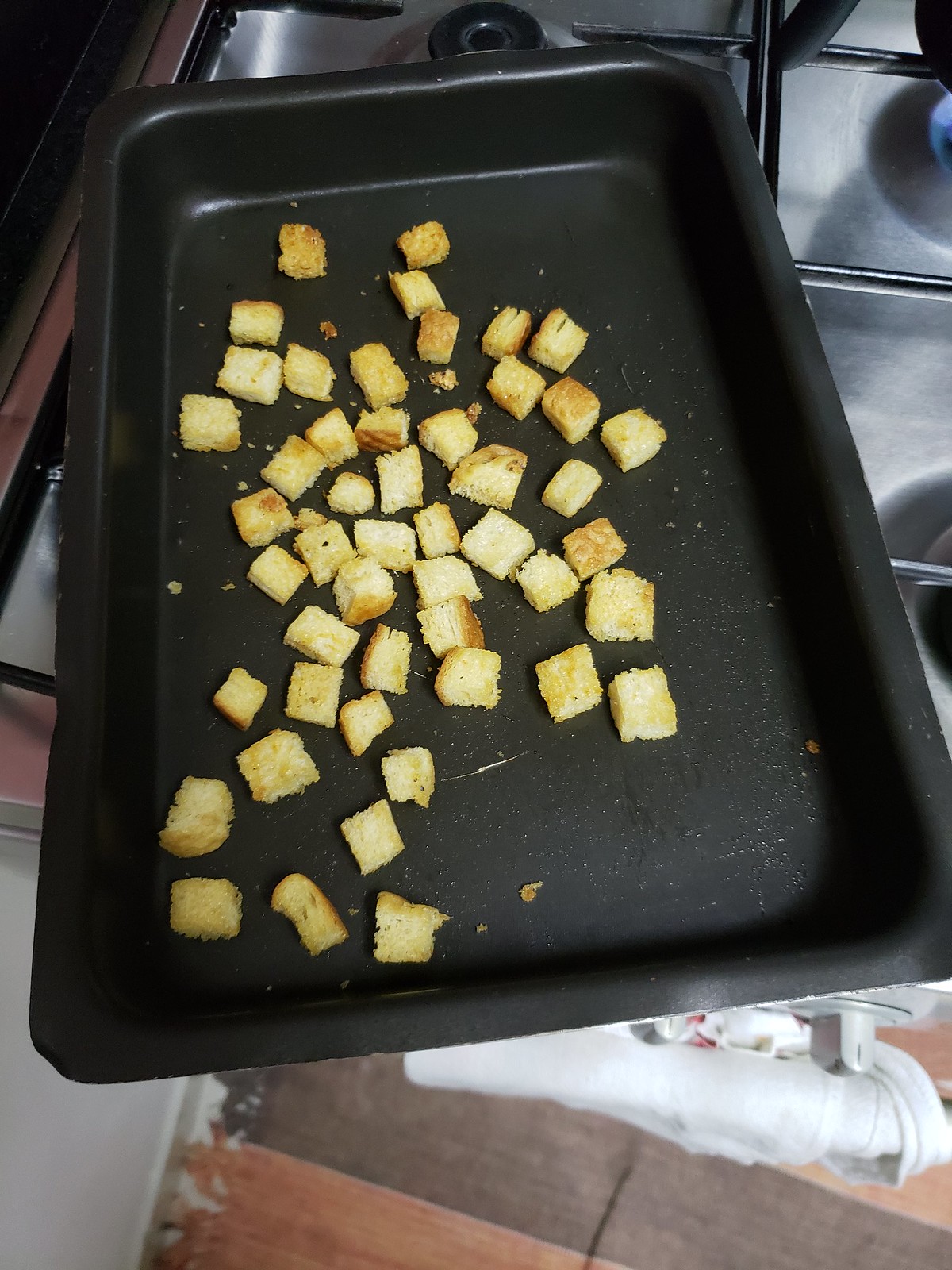The photograph features a gas stove top as the backdrop, with a black, low-profile pan sitting at an angle on the lower left burner. The pan contains golden-brown croutons, neatly cubed and slightly toasted, suggesting they were recently cooked. The gas stove top has white backgrounds around each burner, framed by a cast iron square casing to allow flames to reach the pan. In the bottom right corner, a silver handle, likely for the oven door, can be seen. Additionally, the floor in the bottom of the image displays a pattern of wide planks in alternating shades of maple and dark brown, enhancing the rustic feel of the kitchen setting.